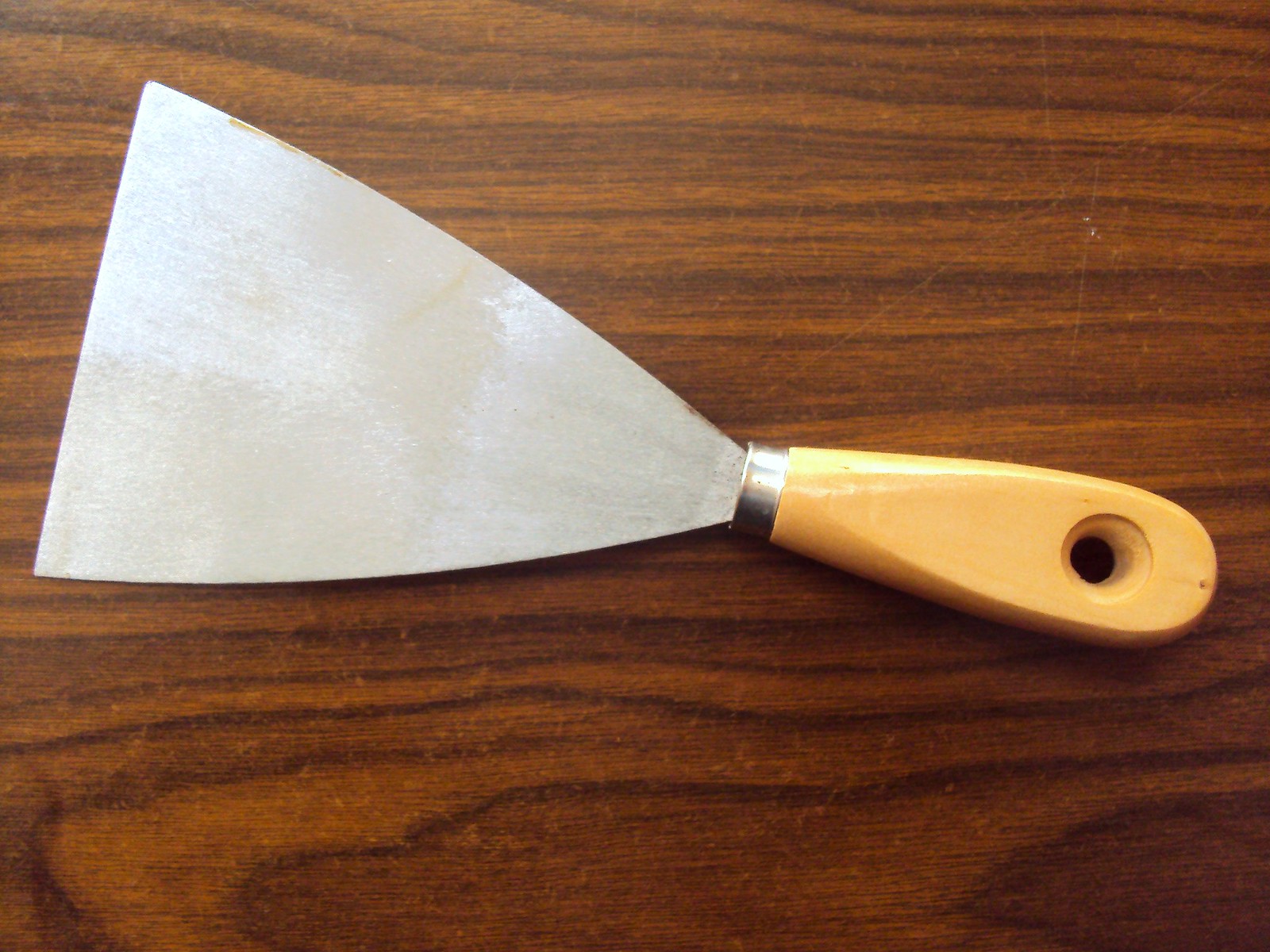The image features a spatula scraper captured from above, with a distinctive triangular metal blade that is widest on the left side and narrows towards the right. The blade is attached to a small, rounded, oval handle, which is yellow and appears to be made of plastic. The handle includes a hole in the middle, designed for hanging. At the top of the handle is a small silver hilt that catches the light, adding a shiny detail to the scene. The metal blade showcases varying shades of silver and gray with some brown marks, indicating usage. The spatula scraper rests flat on a dark brown wooden grain surface, positioned at a slight diagonal.